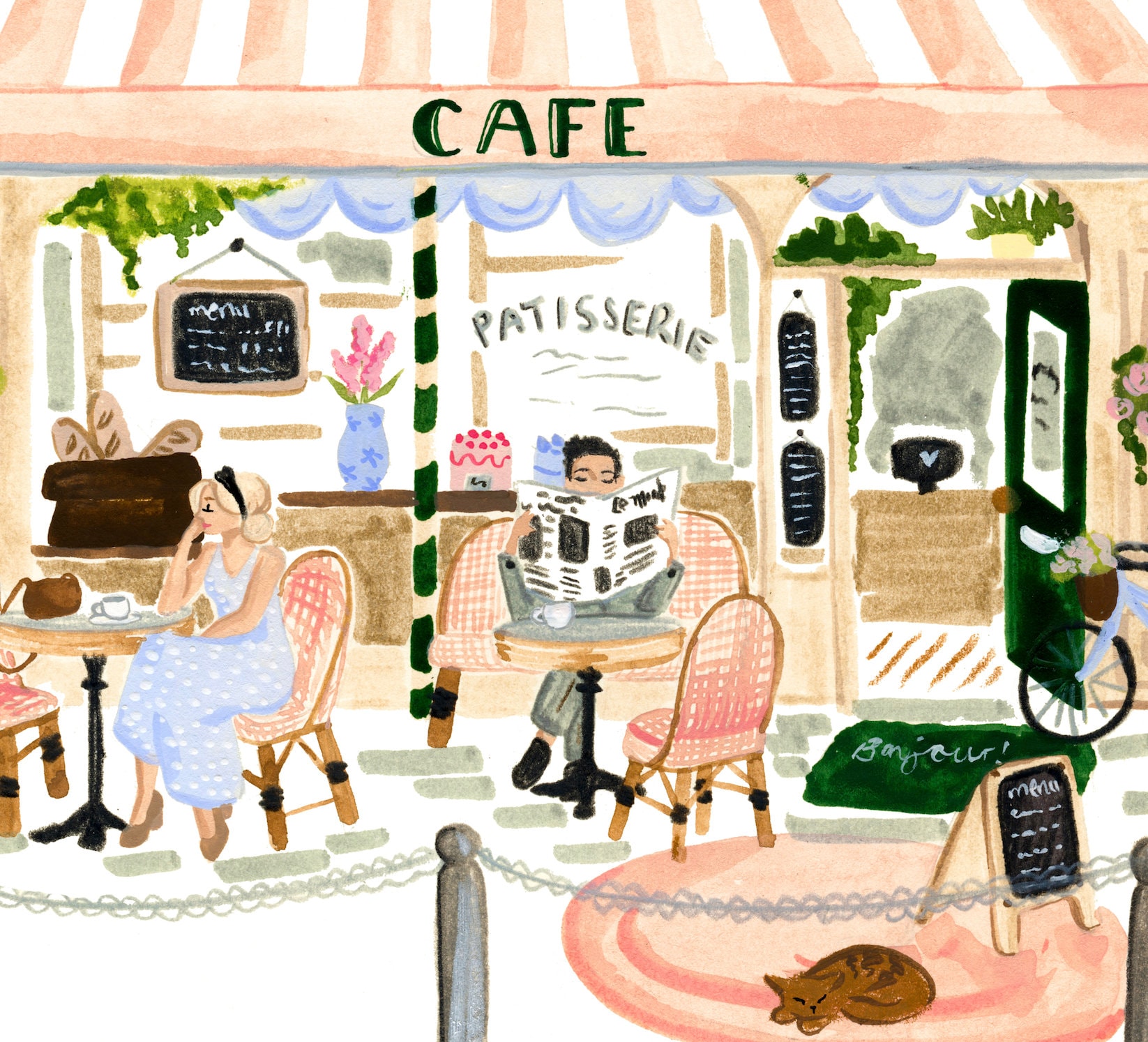The image is a vibrant watercolor painting depicting the cozy exterior of a French café or bistro, adorned with charming details. At the forefront of this inviting scene, under a salmon pink and white striped awning with "Café" written in green letters, two individuals are enjoying their time at separate tables. A wicker bench holds a man sipping coffee while reading a newspaper, identified as "Le Monde." Nearby, a blonde woman wearing a blue sundress and a black headband is also savoring her coffee, her brown purse resting on the table beside her.

The café’s ambiance is enriched by a variety of small yet significant touches: a brown cat sleeps soundly on a pink carpet near the right side, just next to a menu board. The green doormat greeting visitors with "Bonjour" hints at the café's probable location in France. Through the windows behind the man, the word "Patisserie" can be seen, along with a display of baguettes and intricately decorated cakes. A blue vase filled with pink flowers adds a touch of elegance to the window’s decor.

Inside, glimpses of a green door, a cash register, and another menu board complete the picturesque setting. The scene is further animated by the presence of everyday items—a chalkboard menu, baskets of bread, and the hint of a leisurely bike ride indicated by a bicycle near the entrance—exemplifying a quintessential day at a French café.